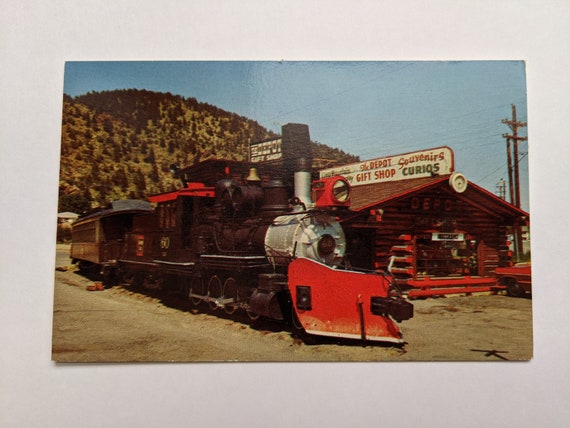This image captures a vintage-style photograph of a black train with a silver nose and a red arch at its front, positioned diagonally to the right on a light brown, barren surface reminiscent of a desert. Behind and to the right of the train stands a rustic wooden gift shop with a white sign that reads "Gift Shop" and "Souvenirs" in red. This small-town scene evokes a western settlement from the late 1800s to early 1900s, further emphasized by green mountains and bushes visible in the background, along with a clear blue sky and some power lines. Just in front of the gift shop, a red car is partially visible. The train consists of the main front car and an additional passenger car, creating a timeless, nostalgic atmosphere.